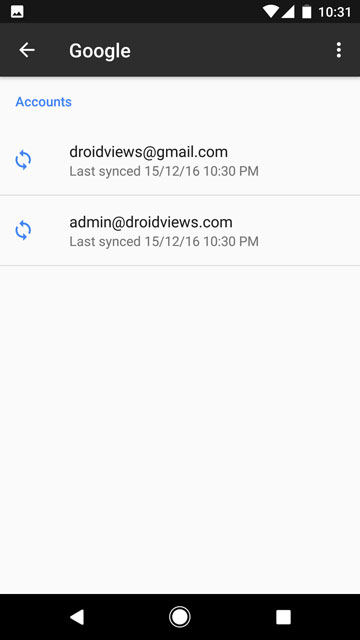This screenshot showcases a user's Google accounts interface. At the top, a black rectangular bar displays the white text "Google" accompanied by a left-pointing arrow. In the top right corner, the current time, "10:31," is visible. Just below this is a menu bar. Beneath it, a white background features the title "Accounts" in blue text.

The main section displays account details. The first entry shows two circular blue arrows to the left, and to the right, "droidviews@gmail.com" with the last sync time noted as "15/12/16 10:30 PM."

Following it, another entry begins with two circular blue arrows to the left, listing "admin@droidviews.com" on the right. This account also has the last sync time recorded as "15/12/16 10:30 PM."

At the very bottom, another black rectangular bar hosts navigation icons: a triangle, circle, and square. This captures the complete layout and details visible in the account management interface.